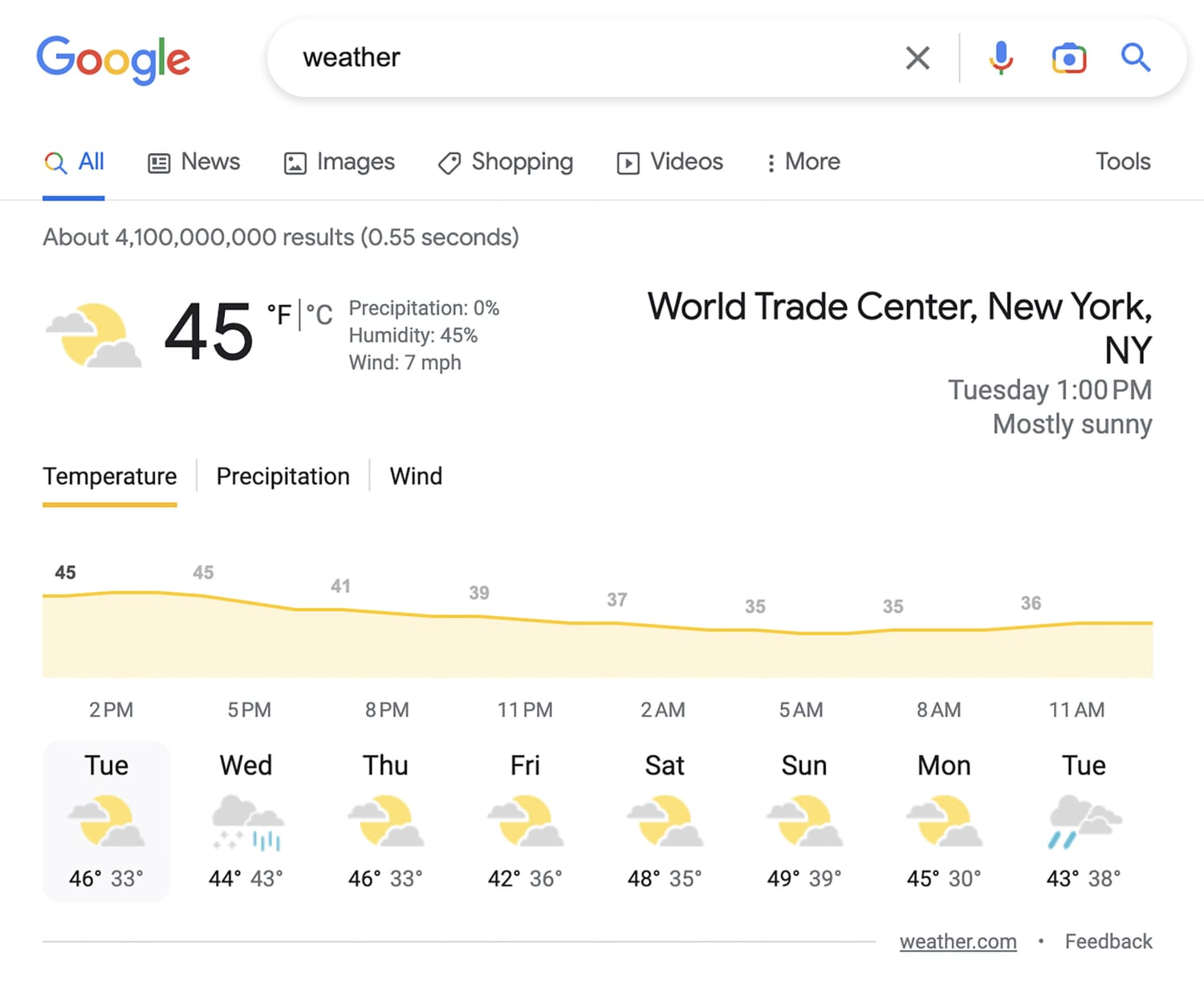The desktop screenshot displayed captures a Google search results page for the query "weather." Although the operating system is not identifiable, several notable elements are present on the screen. At the top, there is a search bar with the typical 'X' for clearing the query, a microphone icon for voice search, a camera icon for image search, and a search icon. Directly above the search results, there are filter options labeled as All, News, Images, Shopping, Videos, More, and Tools.

Google reports approximately 4,100,000,000 results in 0.55 seconds. The weather summary for the World Trade Center, New York, NY at 1 p.m. shows a mostly sunny sky with a temperature of 45°F, which can be converted to Celsius. Additional details include 0% precipitation, 45% humidity, and winds at 7 mph.

Below, a weekly forecast is shown, along with a bar graph visualizing temperature trends from 2 p.m. to 11 a.m. the following day. The forecast highlights are:
- **Tuesday**: Partly cloudy, high of 46°F, low of 33°F.
- **Wednesday**: Rainy, high of 44°F, low of 43°F.
- **Thursday**: Cloudy, high of 46°F, low of 33°F.
- **Friday**: Cloudy, high of 42°F, low of 36°F.
- **Saturday**: Cloudy, high of 48°F, low of 35°F.
- **Sunday**: Cloudy, high of 49°F, low of 39°F.
- **Monday**: Cloudy, high of 45°F, low of 30°F.
- **Tuesday**: Rainy, high of 43°F, low of 38°F.

The source is listed as weather.com, and there’s an option to provide feedback. Overall, the user is searching for weather information in their area using Google.